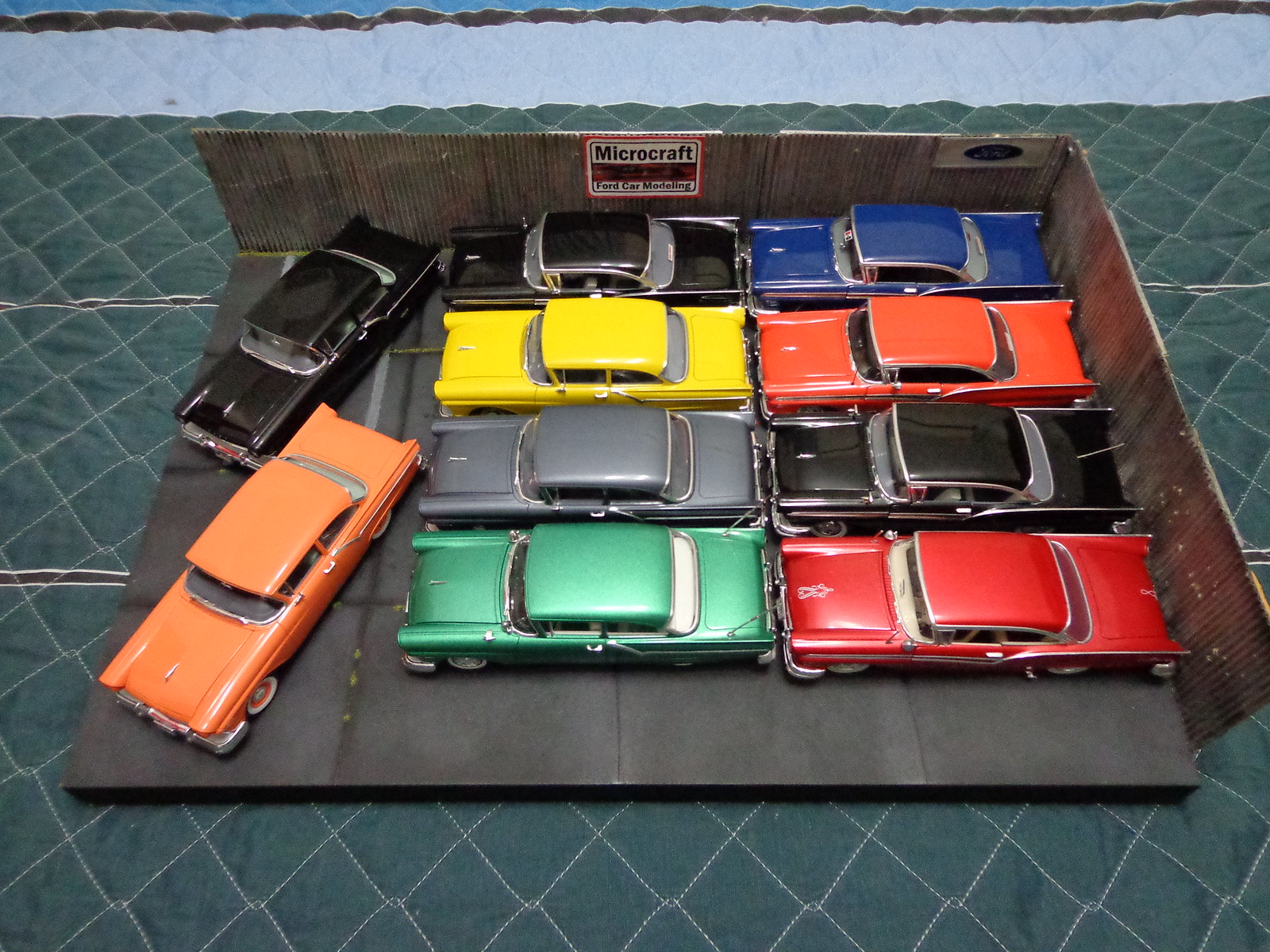The image is a photograph taken from a somewhat bird's-eye view, showcasing a detailed diorama or model scene featuring toy cars. The scene is set on a dark green quilt with a diamond pattern stitched in white, likely laid out on a bed. At the center of this quilt lies a black, open-topped box labeled "Micro Craft Ford Car Modeling," with two sides missing—clearly intended to mimic a garage or car showroom.

Inside the diorama, there are ten vintage-style die-cast toy cars, likely from the 1950s to 1970s, given their rounded fenders and elongated hoods and trunks. Eight cars are meticulously aligned in two horizontal rows, facing left with their tops, roofs, and trunks visible. These cars are colored black, yellow, gray, and turquoise in the first row, and blue, orange, black, and red in the second row. Two additional cars—one black and one dark orange—are positioned at a 45-degree angle to the left of the aligned cars, adding a dynamic touch to the scene. The black box’s surface, resembling asphalt, enhances the look of an actual parking area. The overall effect is reminiscent of a toy car display you might see at a car retail place or in a child's imaginative play setup.